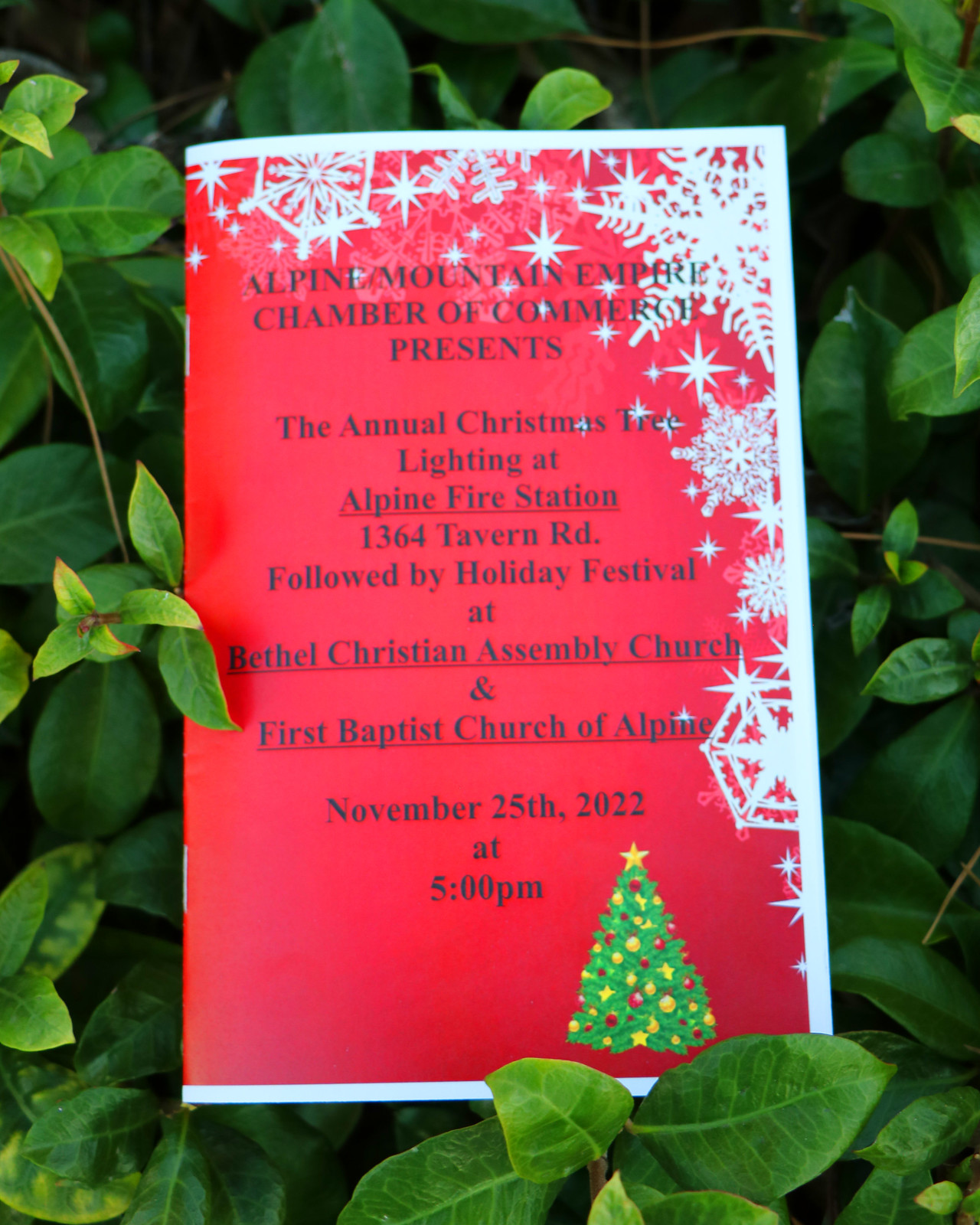In this detailed photograph, a rectangular-shaped paper poster is positioned amid green plant leaves, suggesting it might have been taken outdoors, though the exact setting remains unclear. The poster stands taller than it is wide, resembling the dimensions of a standard 9 by 11-inch booklet. On the left-hand side, visible stapled marks suggest it was part of a bound booklet or pamphlet. The poster features a striking red background with a decorative white border adorned with large snowflakes and small stars on the top and right edges, creating an appearance reminiscent of icy patterns.

Centrally aligned on the poster, black text announces: “Alpine Mountain Empire Chamber of Commerce presents the annual Christmas tree lighting at Alpine Fire Station, 1364 Tavern Road, followed by Holiday Festival at Bethel Christian Assembly Church and First Baptist Church of Alpine.” The event details note it will take place on November 25, 2022, at 5.00 p.m. Additionally, in the lower right-hand corner of the poster, there is a small, festive drawing of a green Christmas tree decorated with a yellow star on top and red and gold ornaments.

The paper poster, encased within a vibrant cluster of green leaves, provides a visually striking contrast and adds a natural element to the festive announcement.